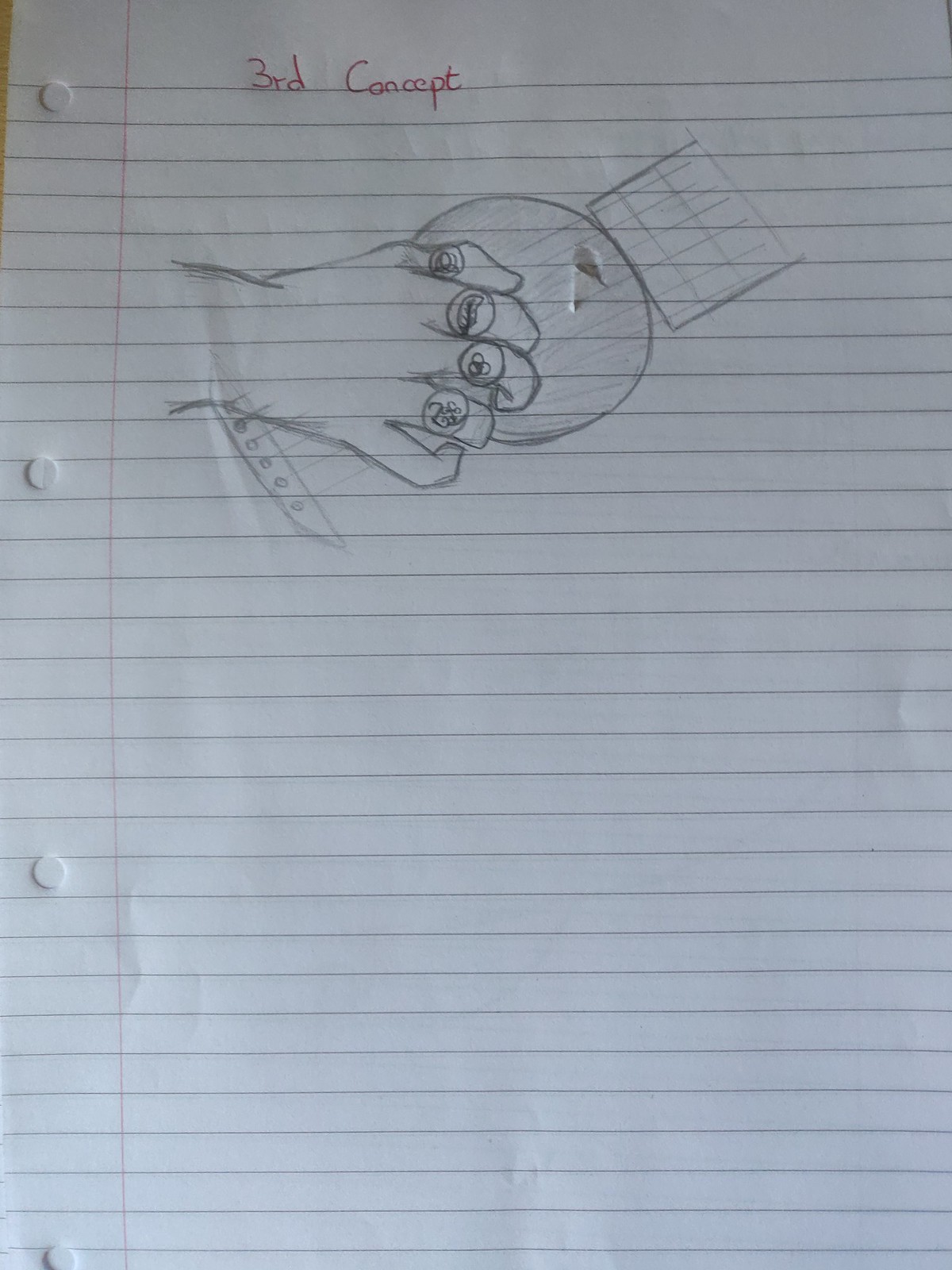The image depicts a sheet of lined paper, featuring dark horizontal lines extending across the entire page. The paper is perforated along the left margin with holes for binder insertion, and the margin is delineated by a red vertical line. At the top of the page, within the thickest section of the margin, the text "3rd concept" is hand-drawn in red ink.

Below this heading, an illustration of a human hand strumming a guitar is prominently displayed. The guitar illustration includes detailed elements such as the bridge, the sound hole, and part of the fretboard. The hand, depicted in the act of strumming, wears rings on the thumb, index, middle, and ring fingers. Each ring is adorned with distinct icons: a feather, three interlinked circles at the center, and two other unidentifiable symbols. The meticulous details and the variety of elements combine to create a visually engaging scene on the otherwise plain sheet of lined paper.